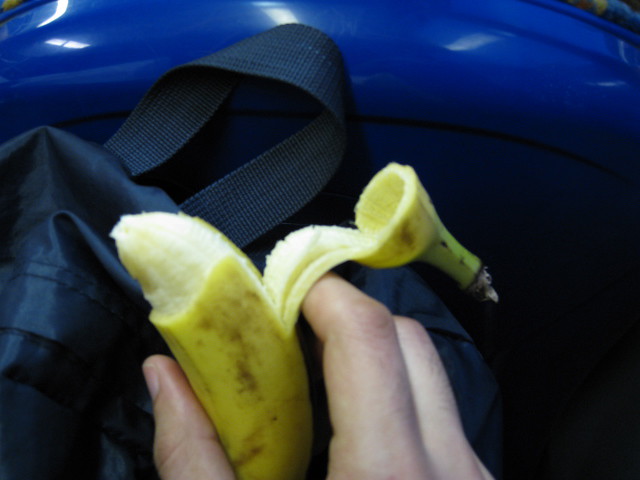This photograph features a detailed close-up of a man's right hand emerging from the bottom of the frame. The skin tone suggests he is Caucasian, and there is a light sprinkling of hair on the back of his fingers. He's holding a freshly peeled banana between his thumb and forefinger. The banana itself is untouched, with the pale, yellowish-white flesh exposed and the bright yellow peel adorned with a few dark spots. The stem of the banana drapes over his index finger where it has been peeled back.

In the background, there's a navy blue backpack, easily identifiable by its zipper and handle crafted from sturdy canvas. The material appears to be waterproof, indicative of its durability. Beyond the backpack, a shiny, hot metallic blue surface with a rounded curvature spans across the top of the image, possibly the roof of a car, adding a reflective and sleek element to the composition.